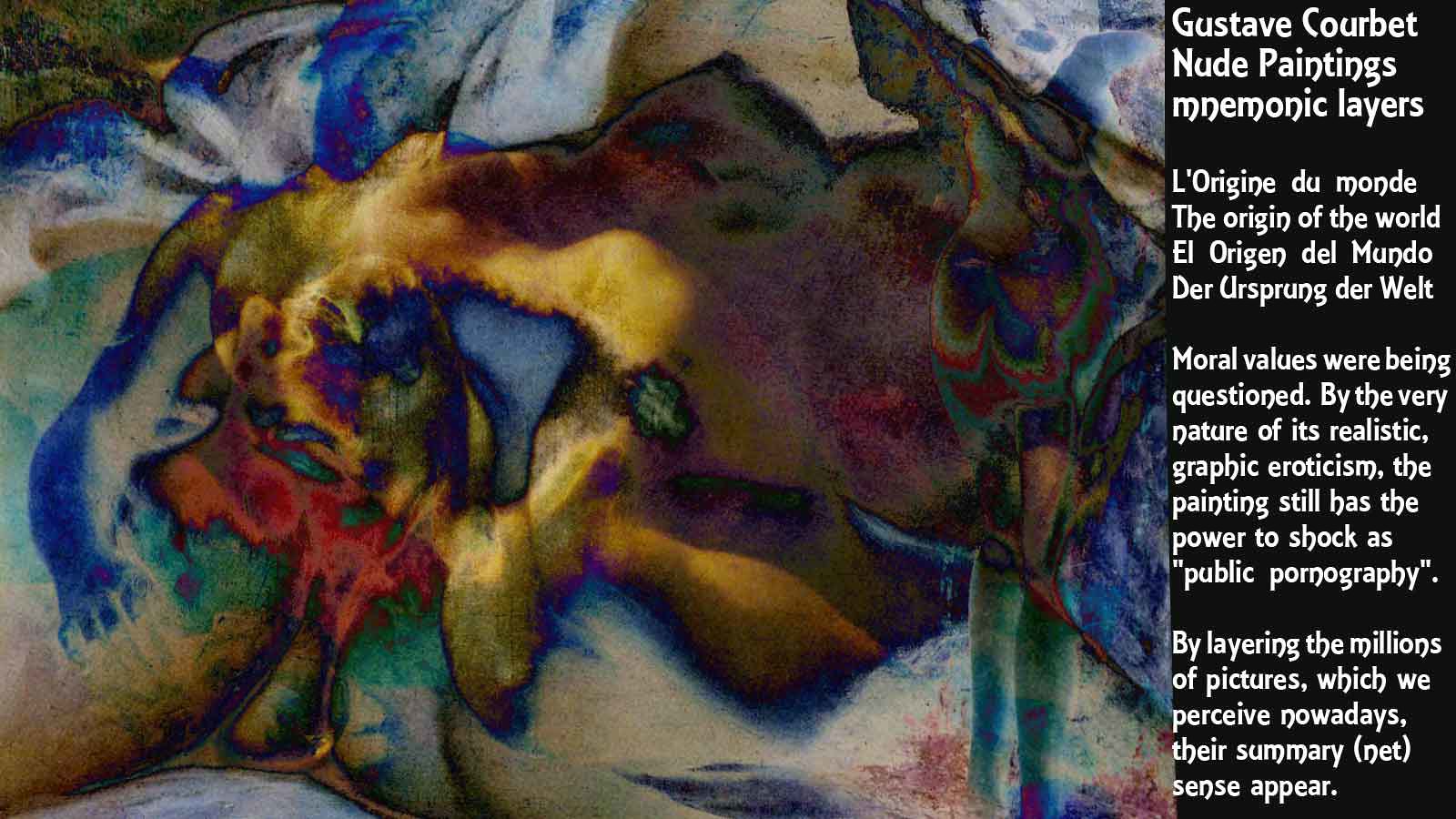The image presents a detailed examination of two distinctive artworks side by side. On the right, there's a painting credited to Gustave Courbet, featuring muted colors with a dark center and interspersed light flesh tones, reds, and blues. Accompanying the painting, a rectangular black background displays text in white that reads: "Gustave Courbet, nude paintings, mnemonic layers." Below this, a paragraph in French precedes an English translation stating, "Moral values were being questioned by the very nature of its realistic graphic eroticism. The painting still has the power to shock as 'public pornography.'" This controversial piece reflects a provocative exploration of moral and social norms through its explicit and realistic depiction.

On the left side, a more abstract and vividly colored artwork portrays a woman appearing to tear her face or chest open, revealing an inner blue background. She extends a bluish arm to the left, while a giant green mole or hole seems to grow around her chest area. The design emphasizes abstract and surreal elements, juxtaposing the raw realism of Courbet's work with a modern, interpretive form. Together, these contrasting artworks invite a conversation about realism, abstraction, and the evolving nature of artistic expression.